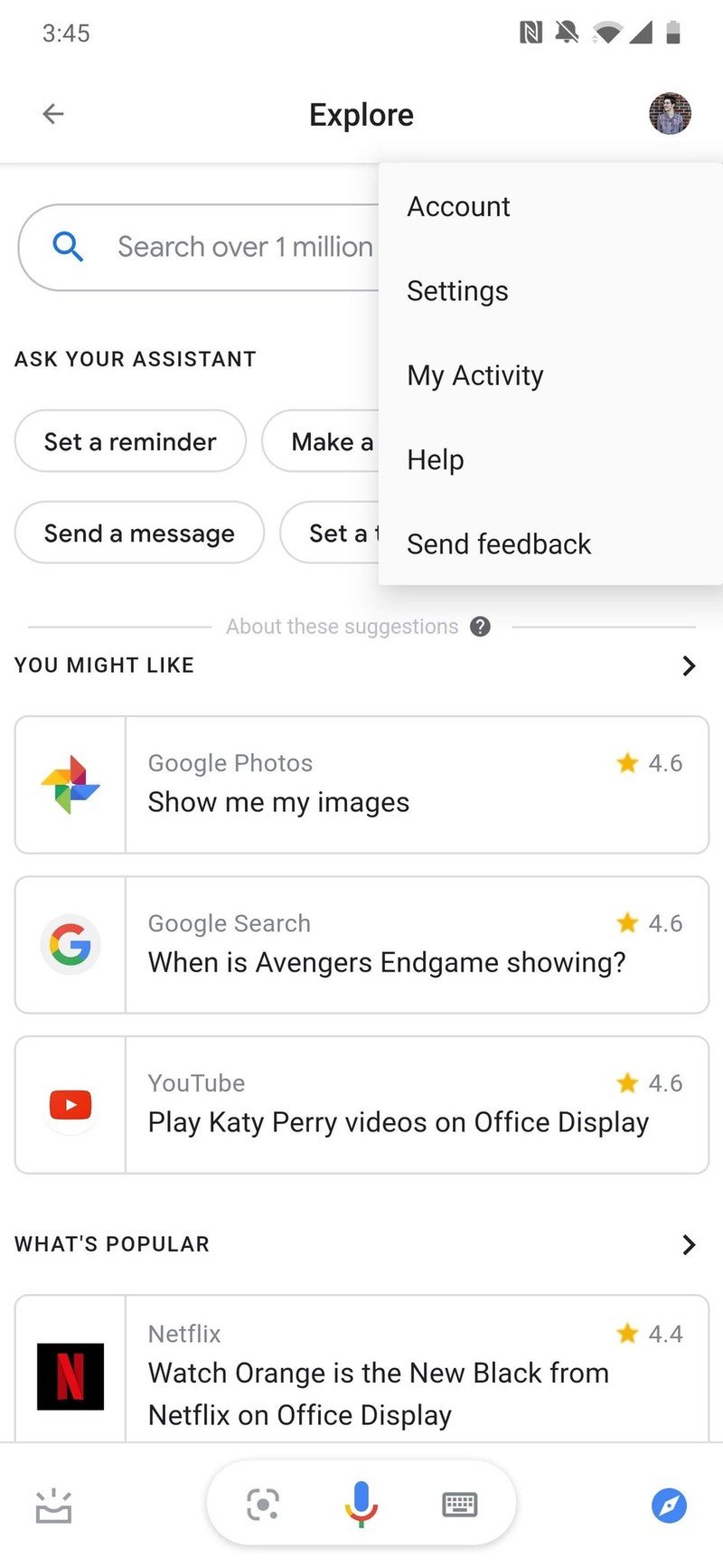This image is a screenshot from a mobile phone displaying a predominantly white interface. The top of the screen shows a gray status bar indicating the time as 3:45, along with several icons: a bell with a strikethrough (indicating silent mode), Wi-Fi signal strength, mobile network signal, and a nearly depleted battery.

Directly beneath the status bar, the screen features a search interface. At the top is a section labeled "Explore" in black font, with an active drop-down menu showing options for "Account settings," "My activity," "Help," and "Send feedback."

Below the drop-down menu, there is a search field with placeholder text that reads "Search for over 1 million." This is followed by black font text suggesting various actions: "Ask your assistant," "Set a reminder," "Send a message," and "Make a set a." Under these suggestions, gray font text reads "About these suggestions?" with a question mark symbol indicating further information is available.

Continuing down the screen, a heading in black font states "You might like," followed by three rectangular selections:
1. "Google Photos: Show me your images" with a rating of 4.6 stars.
2. "Google Search: When is Avengers Endgame showing?" also rated 4.6 stars.
3. "YouTube: Play Katy Perry videos on office display," likewise rated 4.6 stars.

At the very bottom, under the heading "What's popular," another gray rectangle suggests "Netflix: Watch Orange is the New Black from Netflix on office display."